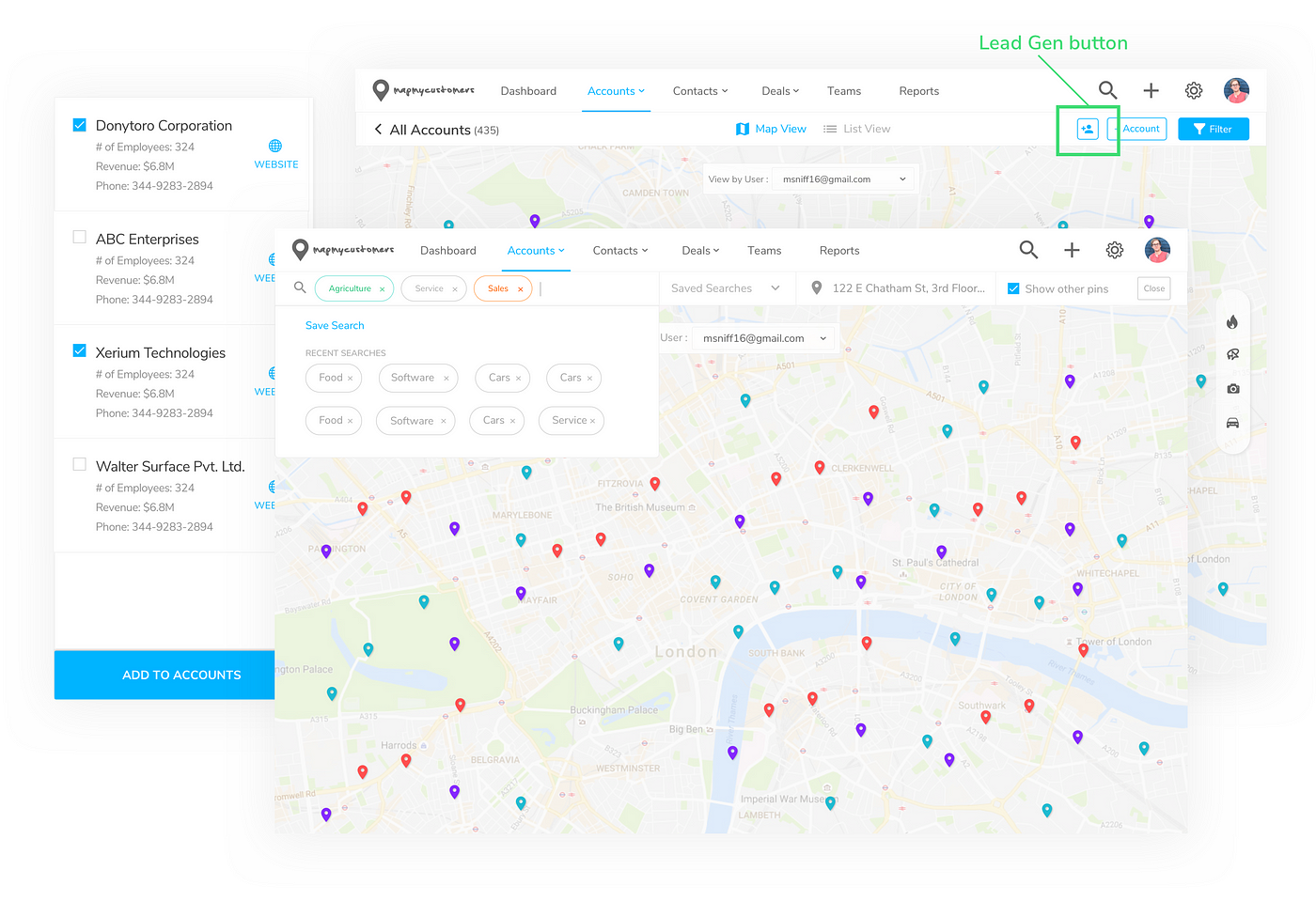The image is a horizontally rectangular screenshot showcasing a digital interface. Dominating the right side of the image is a white vertical rectangle featuring a list of different locations, two of which are marked with checkmarks. At the bottom of this vertical box, a prominent blue button labeled "Add to Accounts" is clearly visible.

In the upper section of the image, there is a white horizontal banner containing various tabs labeled "Dashboard," "Accounts," "Contacts," "Deals," "Teams," and "Reports." To the right of these tabs, an "Add a Person" icon button, outlined in green with a slight diagonal line extending from the top center to the left, is present. Directly above this icon, a green "Lead Gen" (Lead Generation) button is positioned.

The main background of the image depicts a map filled with an abundance of various colored points, including red, purple, and teal. Additionally, there is another smaller window, also showing a map, which has popped up over the main map, further contributing to the visual complexity of the image.